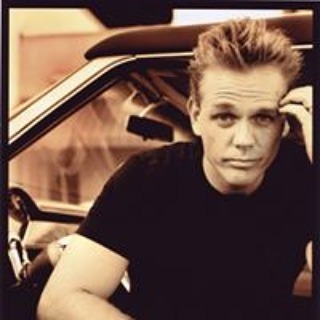In this evocative sepia-toned photograph, a man with long hair sits pensively in the driver's seat of a car with the door open. He is dressed in a black shirt, and his right hand rests thoughtfully on his head. The image exudes a nostalgic and introspective atmosphere, reminiscent of an album cover, yet the identity of the individual remains unknown, adding an element of mystery to the scene.